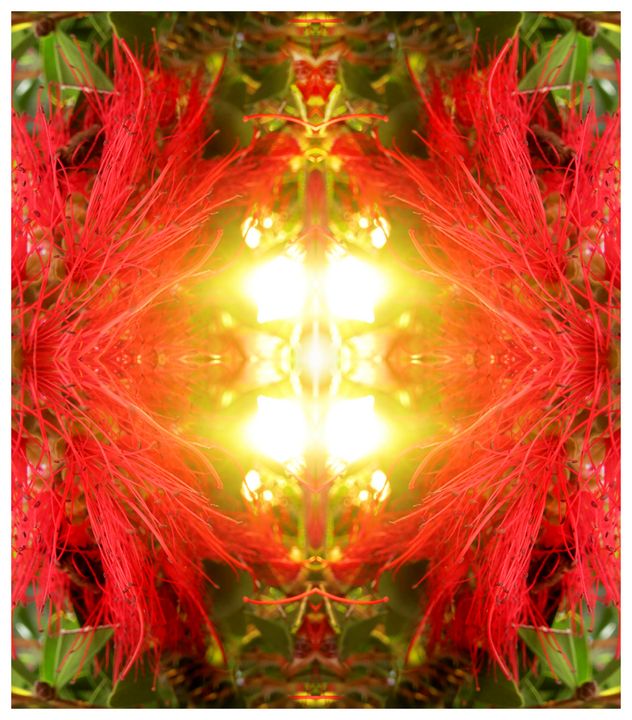The image is a square, abstract piece featuring a vivid, kaleidoscopic design. At its center is a glowing, vertically-oriented rectangular light emitting a bright white and yellowish hue. This radiant core is flanked by grouped, thin red stems that converge, creating an open pathway that allows the light to shine through. Surrounding the luminous center are intricate, interconnected red branches. At both the top and bottom of the glowing light is a long, skinny face with its mouth open, emitting the same white or yellow light. Notably, the bottom face appears upside down, giving a mirrored effect.

The entire composition has a surreal, almost hallucinogenic quality, with the top and bottom halves of the image appearing as mirror reflections of each other, as do the left and right sides. The periphery of the image features green leaves shaped like upside-down triangles, with their wide ends pointing upwards, adding to the image's symmetrical and trippy aesthetic. The combination of bright red stems, glowing yellow and white light, and lush green leaves against the symmetrical design creates a dynamic and visually captivating artwork.